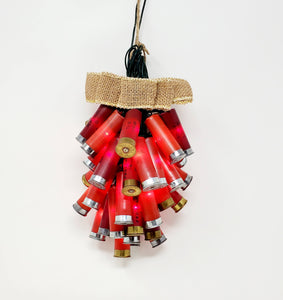In this image, a unique Christmas decoration hangs suspended against a plain white background, its shadow softly mirrored on the surface. The centerpiece of this creation is a cluster of red shotgun shells, arranged artfully to resemble a bouquet or the shape of a pine cone. Each shell glows with a red light from within, emphasizing their cylindrical form. They are held securely by a burlap ribbon, adding a rustic charm. This ribbon ties the shotgun shells together in a dense grouping at the top, which gradually tapers down towards the bottom. The shotgun shell casings are capped with mixed tones of bronze and silver at their bases, adding a contrasting detail. The overall effect is both striking and intricate, giving a creative twist to traditional holiday decor.